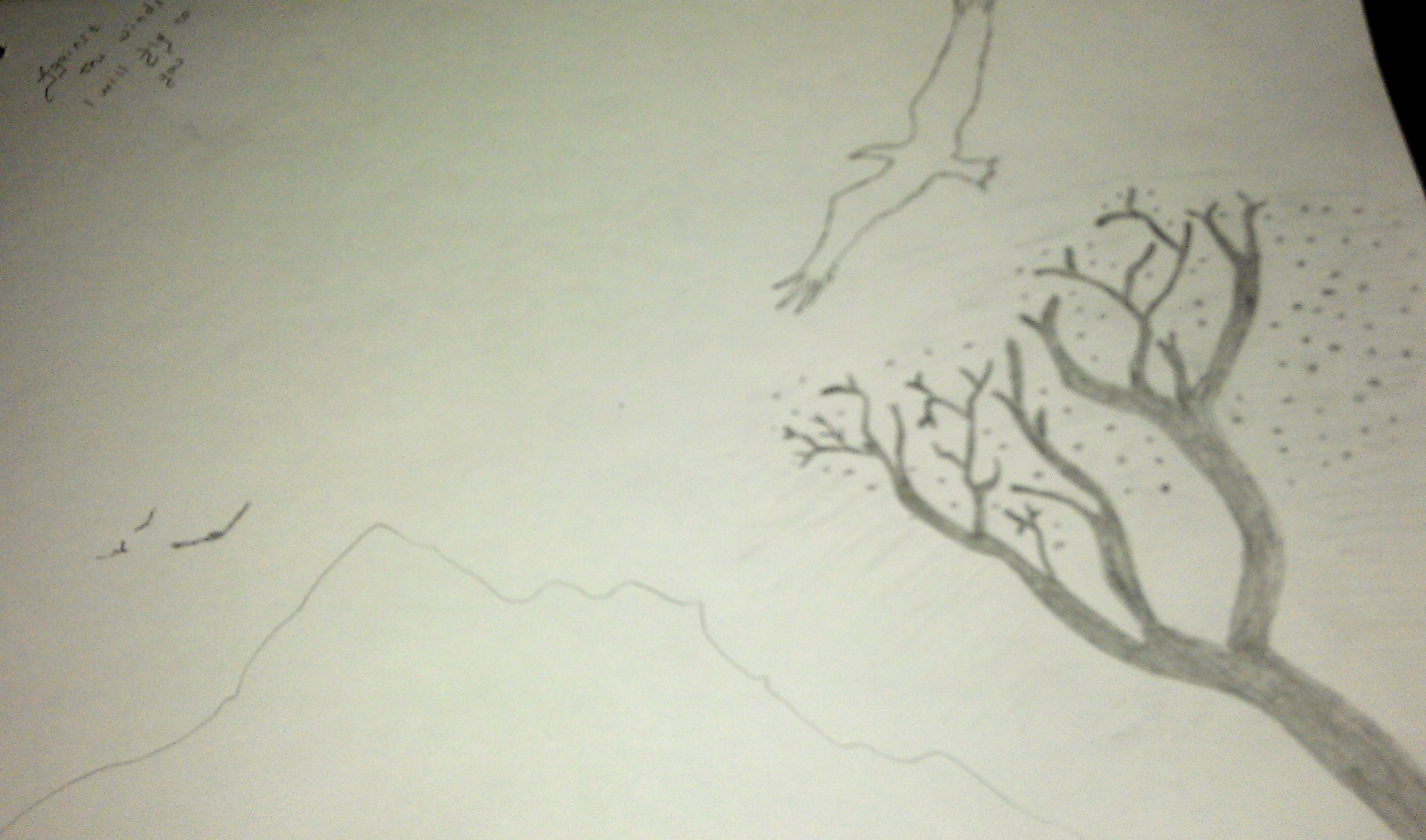This image captures a detailed pencil sketch on a piece of cream-colored paper, possibly from an art journal. Dominating the scene is a large bird, likely an eagle, gliding majestically across the sky with its wings fully stretched out. In the lower right corner, a tall, multi-branched tree is depicted, with leaves blowing off into the wind, represented by a myriad of black dots. At the center bottom of the image, an outline of mountains serves as a serene backdrop. Several smaller birds, perhaps blackbirds, are flying in the distance over the mountain range. There is also some handwritten text in the upper left corner, adding a personal touch, though it remains illegible. The image appears slightly skewed, enhancing the feeling of a candid, in-progress sketch from an artist’s perspective.